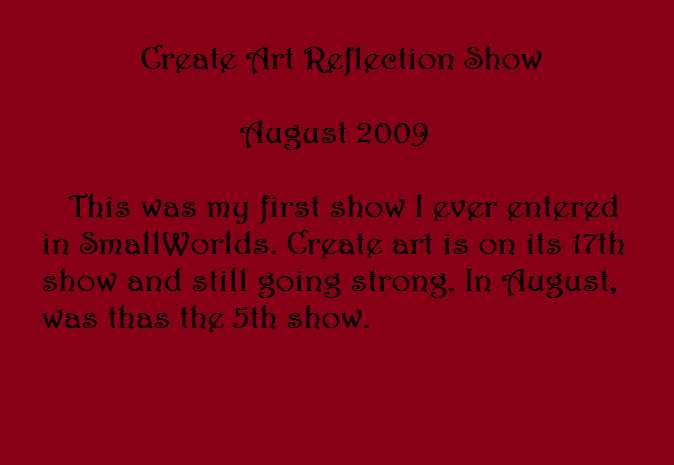Here we have a digitally generated image featuring an announcement on a bright red background with vivid black text in an exaggerated, creative font. At the top, the bold headline reads "Creative Art Reflection Show," each word capitalized. Below, there's a gap followed by "August 2009." Further down, a paragraph reads: "This was my first show I ever entered. Create Art is on its 17th show and still going strong. In August, this was the fifth show." The unusual font adds a distinctive flair to the text, with letters like the 'S' curling in on themselves. The rest of the image is simply the red background with no additional elements.